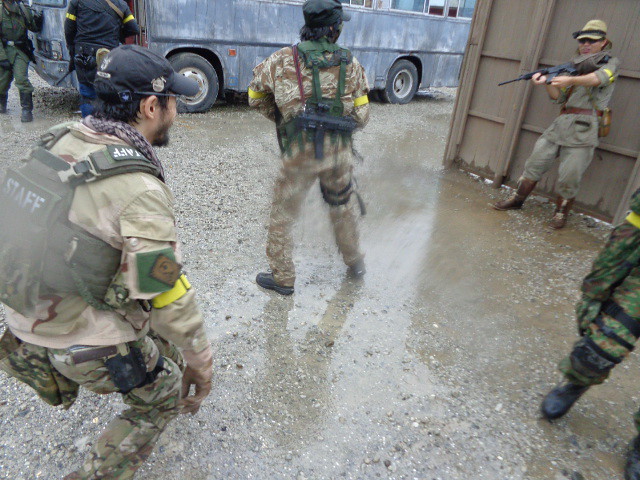The photograph depicts what appears to be either airsofters or soldiers standing on a rain-soaked gravel and mud ground dotted with dark brown puddles. In the background, a weathered bus, which might have once been white but now has gray, faded paint and flat rubber tires with white rims, is visible. All the bus's windows and its door are open. 

To the right of the image, a brown plank fence can be seen, against which a person in a gray-brown uniform, brown leather belt, brown leather boots, and a brown hat, is leaning. This individual is holding an assault rifle. In front of him, another man dressed in brown camouflage, with an assault gun strapped to his back, and wearing a green hat is noticeable.

To the left of this person stands another individual wearing camouflage pants, a brown tan shirt, and a blue hat. He has brown hair, facial hair, and a strap across his back labeled "staff." At the far right, just partially visible, is a person dressed in green camouflage, identifiable only by his black-booted leg, gloved hand, and matching camouflage attire. In the background, near the bus, two people in black shirts and black pants are also present.